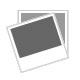This black-and-white photographic image captures a moment outdoors during the daytime, showcasing a soccer team in two rows, set against a gray, cloud-filled sky and a grassy field. The photo, encased in a light brown wooden frame, has a classic, monochrome aesthetic that lends a timeless quality to the scene.

In the back row, six individuals stand with their hands positioned behind their backs. Five of these standing members, donning dark and gray striped jerseys, are players. Positioned next to the fifth player on the left, a man dressed in a sweater and collared shirt, likely the coach, adds a contrasting note to the team uniform.

Kneeling in the front row, five more players add dimension to the composition. Significantly, one player on the far left is black, while the remaining individuals, including those in the back row, are white. Prominently, the player in the center and the player at the far right of the kneeling row each have a soccer ball resting under their right hand.

In the background, a few indistinct signs, displaying only partially visible letters "S" and "EX," along with a spectator stand, hint at the lively atmosphere during the moment of capture. The detailed depiction of the team's arrangement, combined with the evocative outdoor setting, provides a compelling snapshot of the soccer team's posed readiness.